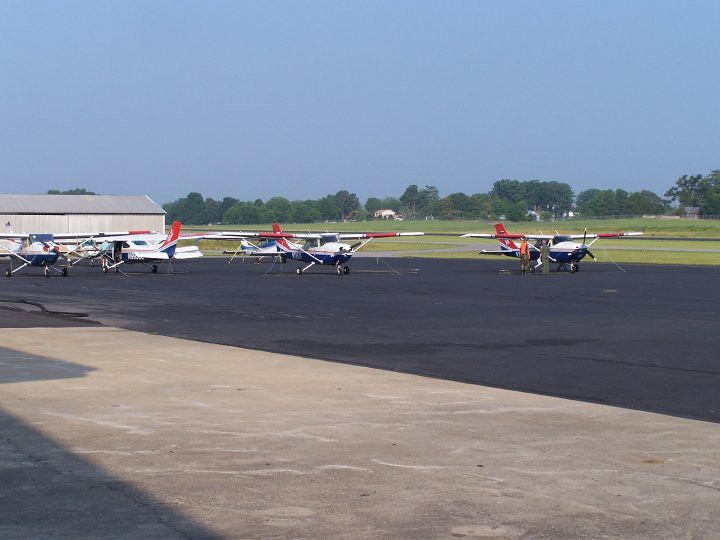This detailed photograph captures a sunny daytime scene at a rural, private airport for small planes. The central feature is a wide, asphalt tarmac strip that accommodates multiple single-engine Cessnas, which appear to be business-related, perhaps for a flight school or a fly-in event. There are five planes visible in the foreground, all similarly marked with a white top half, blue bottom half, white wings with an orange section, and a tail tip that is orange with a white horizontal stripe and blue beneath it. To the left, a barn-like hangar stands adjacent to the blacktop and concrete apron of the staging area. In the background, a grassy field and distant trees border the scene, with a few scattered houses visible far off. Additionally, two individuals stand near the plane on the far right, one dressed in orange and the other in green, engaged in conversation. The sky above is a vibrant blue, further illuminated by the shining sun.